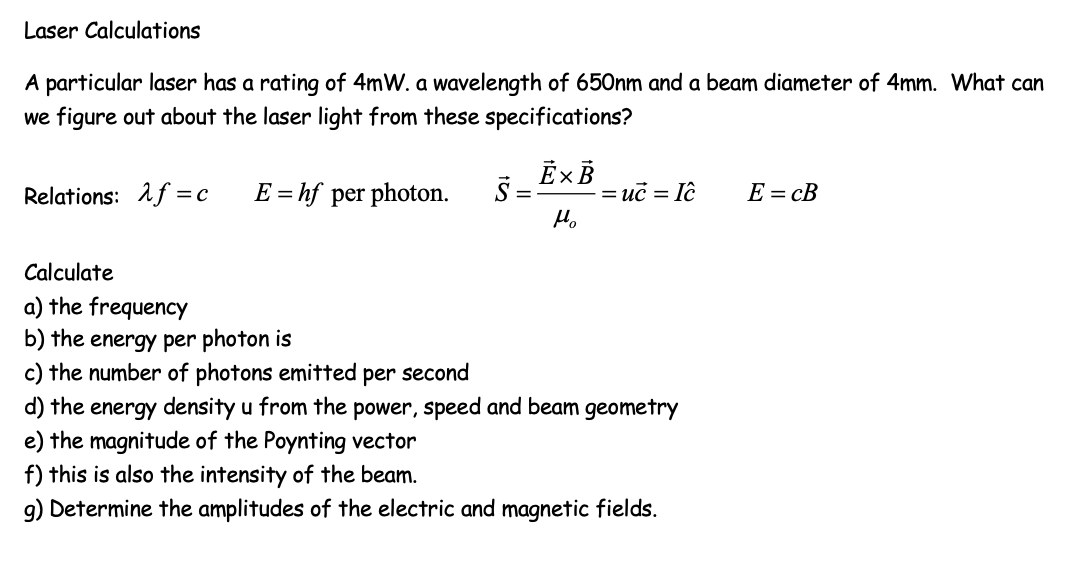This image illustrates a detailed math problem involving calculations with lasers. The laser in question has a power rating of 4 milliwatts, a wavelength of 650 nanometers, and a beam diameter of 4 millimeters. Using these specifications, several physical properties of the laser light are to be determined. The related equations include frequency (ν) calculation using \(ν = \frac{c}{λ}\) and energy per photon (E) using \(E = hν\). Further steps involve calculating the number of photons emitted per second, the energy density (U) from the power, speed, and beam geometry, the magnitude of the Poynting vector \( \vec{S} = \vec{E} \times \vec{B} \) with its directional components, and finally, determining the amplitudes of the electric (E) and magnetic (B) fields. The problem sets a clear path from determining the fundamental properties of laser light to computing complex vector magnitudes and field amplitudes, underlining a comprehensive approach to understanding laser physics.